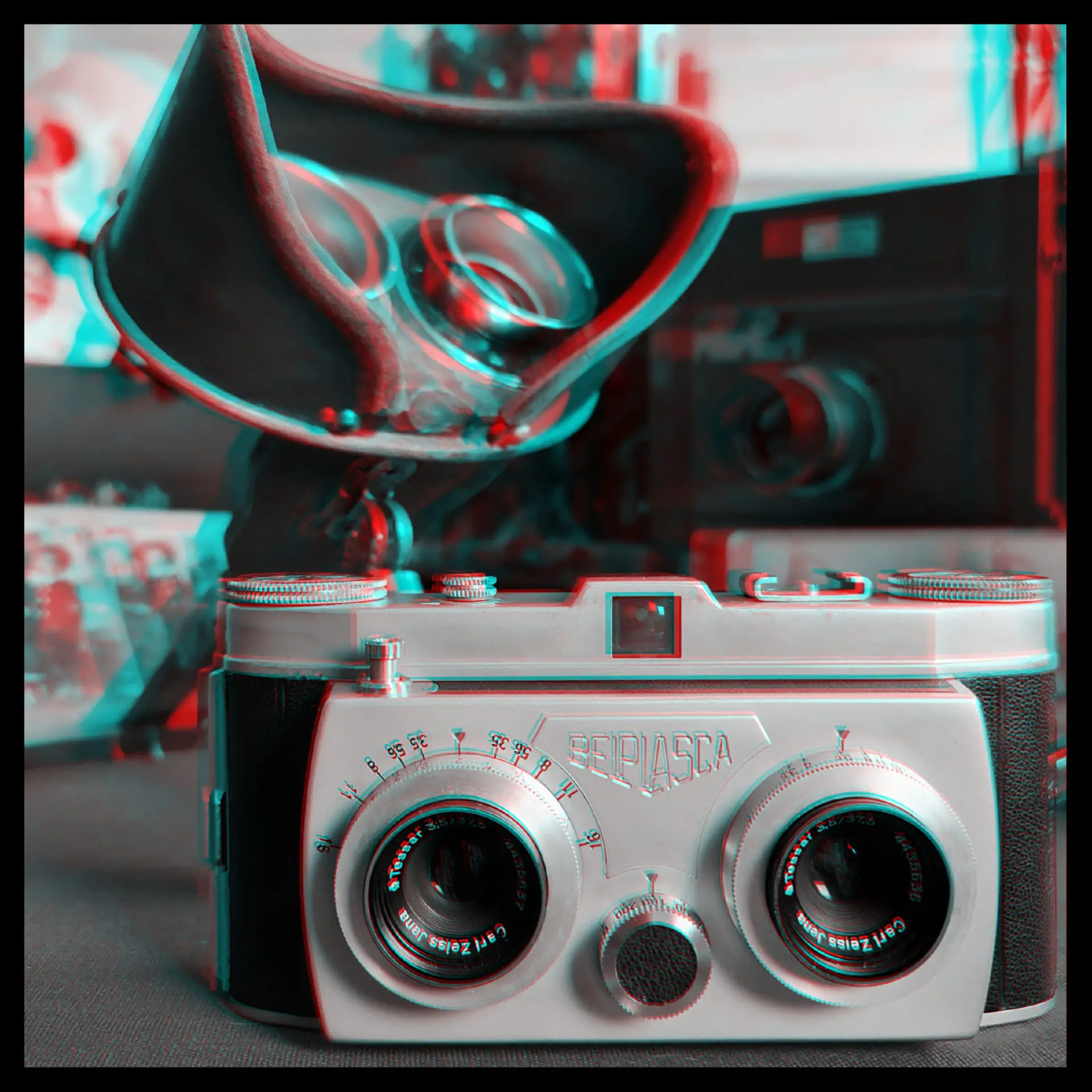The image is a blurred Polaroid photo with a characteristic black border surrounding it, taken indoors with a distinctive blue and red filter applied, giving it a 3D effect. The focal point is an antique camera, prominently featuring two black lenses. Each lens is surrounded by metallic dials displaying various numbers such as 35, 8, 5, 11, and 16, indicating adjustable settings. Central to the camera is another metallic knob, hinting at its intricate functionality. The camera's body combines metallic elements with black leather sections, suggesting durability and vintage charm. Notably, the camera bears the label "Sepp Osaka," though the text is somewhat illegible. Behind the camera, the image reveals additional photographic equipment, potentially including other cameras or record players, along with some prints leaning against a wall. The scene is set on a dark, charcoal-gray surface, adding to the nostalgic ambiance of this visually intriguing shot.